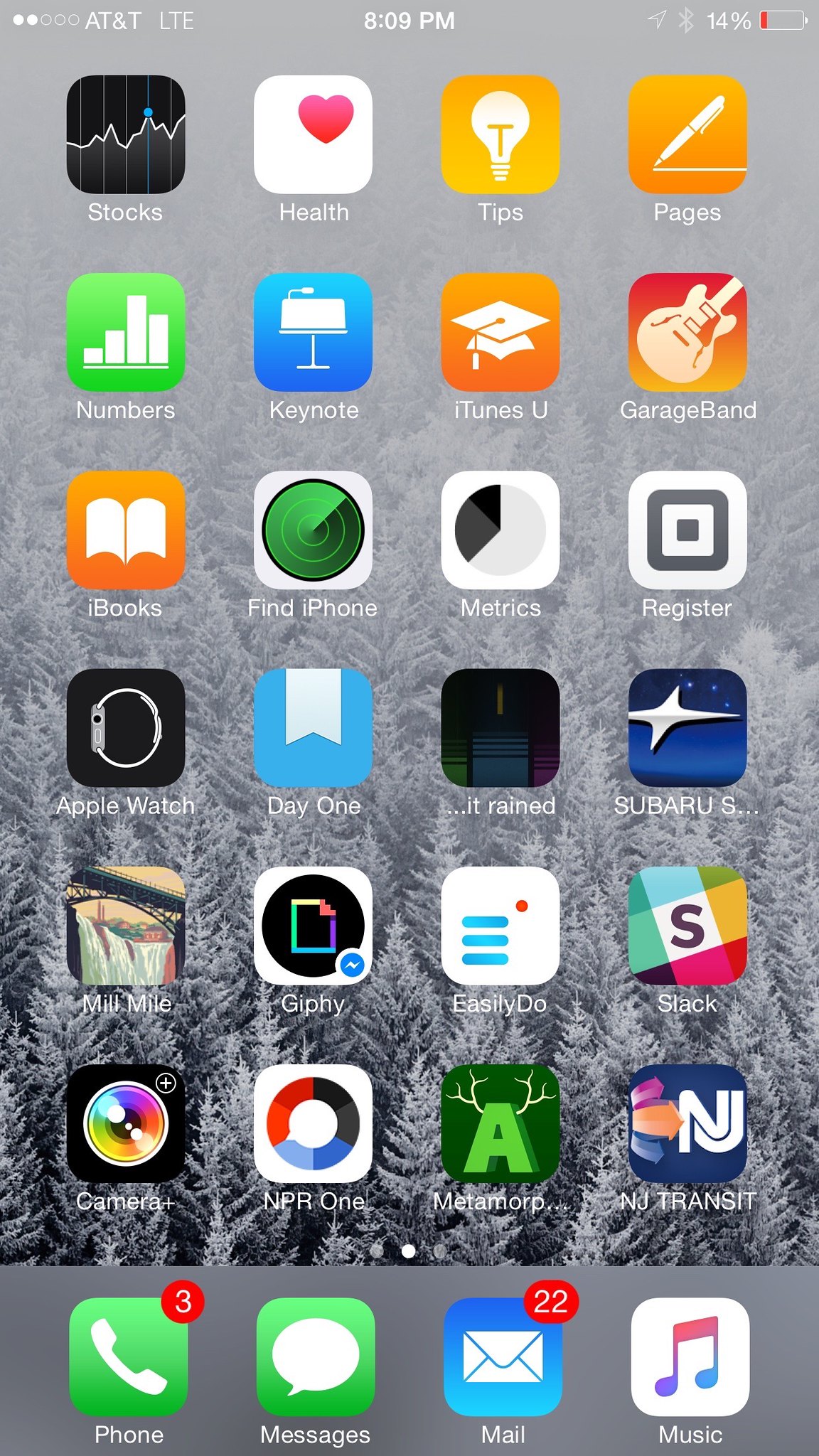This is a detailed screenshot of an iPhone home screen. At the top left, the status bar indicates the device is connected to AT&T with LTE signal strength. The time reads 8 or 9 p.m., and the battery icon to the right shows 14% remaining battery life, depicted in red.

Underneath the status bar, a colorful array of app icons is displayed. From left to right, the icons presented are as follows:

1. **Pages**: An orange square featuring a white pen and line.
2. **Tips**: An orange square with a light bulb icon.
3. **Health**: A white square with a red heart.
4. **Stocks**: A black square with a blue circle containing a squiggly line and dot.
5. **Numbers**: An app icon consisting of four green grid squares varying in size.
6. **Keynote**: A blue square with a podium and microphone illustration.
7. **iTunes U**: A blue square with a graduation cap.
8. **GarageBand**: An orange square with a white guitar.

Below the first row are the subsequent icons:

1. **Register**: A white square with a gray square inside another white square.
2. **Metrics**: A white circle partially covered by a black half-circle.
3. **Find iPhone**: A green circle with a bullseye graphic.
4. **iBooks**: An orange square featuring a white book icon.
5. **Apple Watch**: A black square with a white watch icon.
6. **Day One**: A blue square displaying a white flag or ribbon.
7. **It Rained**: A black square showcasing green, blue, and pink bars.
8. **Subaru**: A blue square with the white Subaru logo.

Further down, there are more app icons:

1. **Slack**: A square with a checkered pattern of blue, green, yellow, and pink with an "S" in the center.
2. **EasilyDo**: A white square with blue lines and a red circle.
3. **GIPHY**: A white square containing a black circle with a multicolored square.
4. **MileMyMile**: An icon displaying a bridge over water.
5. **Camera**: A black square with a camera lens icon.
6. **NPR One**: A white square with a tricolored circle in red, black, and blue.
7. **Metamorph**: A green square with a green "A" and antlers.
8. **NJ Transit**: A blue square bearing the initials "NJ" in white, featuring purple, orange, and blue diamond-like patterns.

The final row of icons includes:

1. **Music**: A white square with a music note.
2. **Mail**: A blue square with a white envelope, showing a red circle with the number 22.
3. **Messages**: A green square with a speech bubble icon.
4. **Phone**: A green square with a phone icon, showing a red circle with the number 3.

Each app icon is distinctly designed, providing a clear visual reminder of its function, ensuring the user is well-versed in quickly finding and accessing each application on their device.